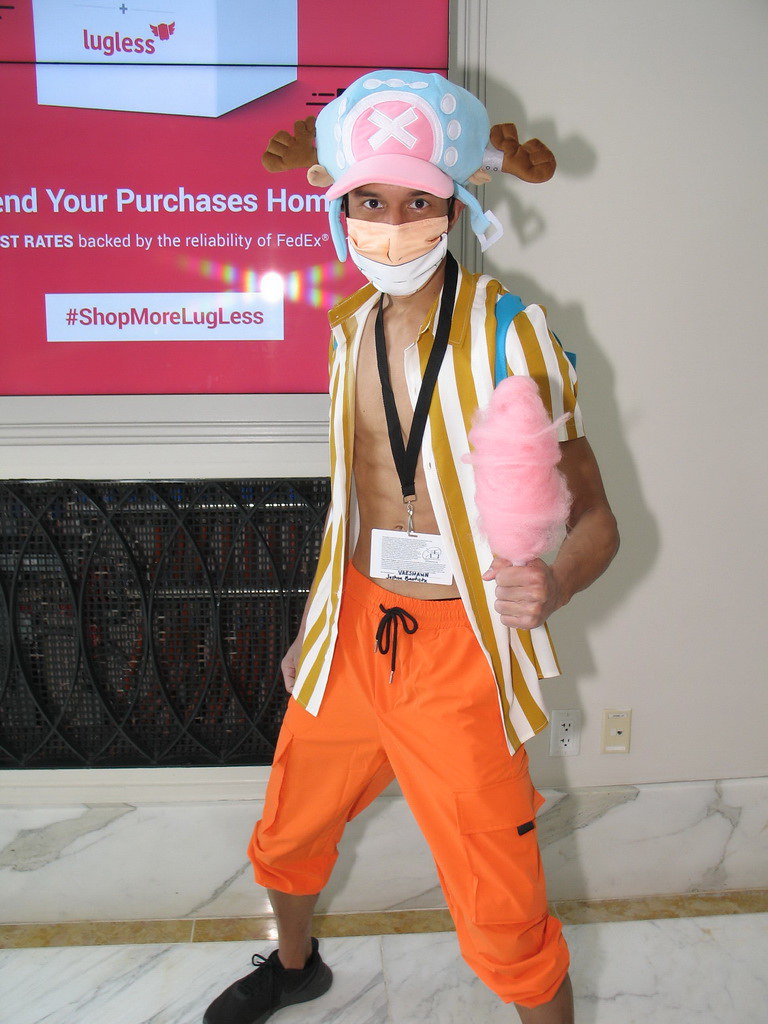In this vibrant photograph, a young boy stands confidently, capturing the viewer's attention. He is dressed in an open, orange, and white short-sleeved shirt that exposes his chest and stomach, paired with bright orange pants resembling those you might find in a karate studio. On his head rests a whimsical pink and blue cap adorned with cartoonish bull-like horns on either side, adding a playful touch to his appearance. His face is partially obscured by a pink and white mask, suggestive of a COVID precaution. 

In his left hand, he griped a fluffy cone of pink cotton candy, and around his neck hangs an ID lanyard that extends all the way down to his waist. A white strap, likely part of a backpack, crosses over his left shoulder. The image features him positioned against a white wall adorned with a pink background poster, promoting a product called "Lug Less." The poster includes the slogans "take your purchases home" and "#shopmorelugless." Below the poster is a black metallic vent. The ground beneath him is made up of intricately designed white tiles. Staring straight into the camera from a slightly crouched stance, the boy exudes a mix of charm and boldness that makes the photograph captivating.